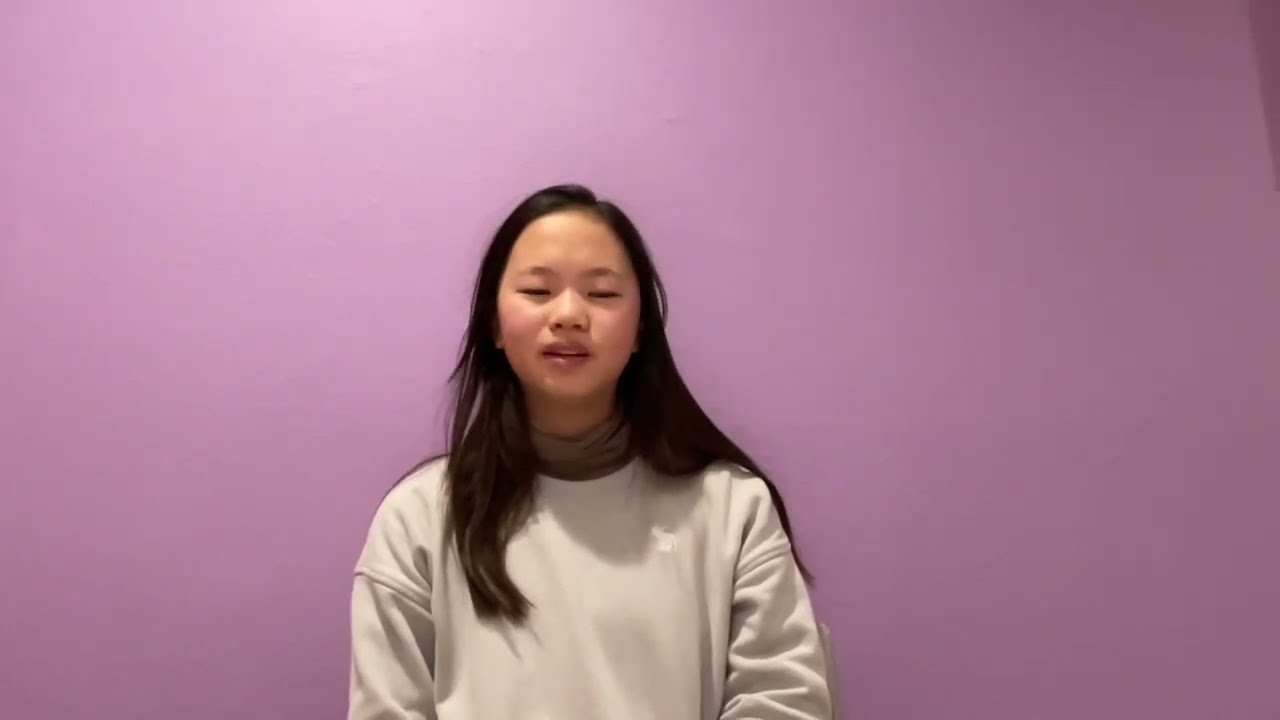This landscape-style photograph captures a young woman of Asian descent standing against a light lavender wall, which serves as the entire background. The wall features darker portions on the right side, illuminated by overhead lighting that casts subtle shadows. The woman appears to be mid-sentence, with her mouth slightly open and her eyes closed, possibly mid-blink. Her long black hair flows down on both sides, with one side draped over her shoulder and torso, while the other side cascades down her back. She is dressed in a cream-colored sweatshirt featuring an indistinct white emblem on the top left, and underneath, she wears a layered grayish or mauve turtleneck. The image, taken indoors, depicts a realistic and representational scene with no additional objects or text in the frame, suggesting she might be recording a video or giving a presentation.